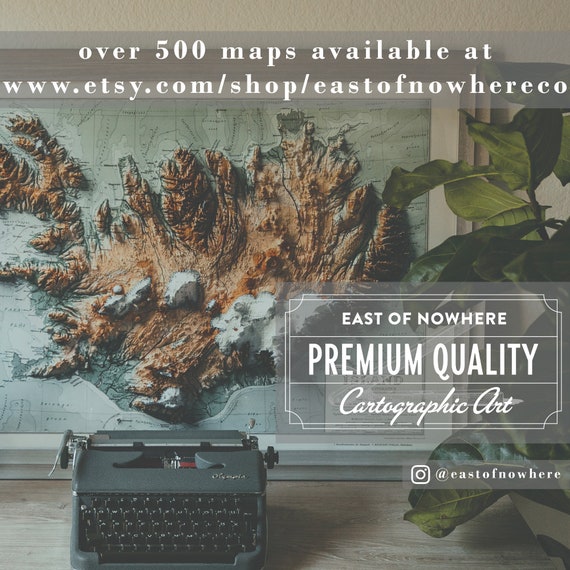This image appears to be an advertisement for East of Nowhere Co., showcasing their premium quality cartographic art available at www.etsy.com/shop/eastofnowhereco. Prominently featured at the top is the text "Over 500 maps available," followed by the web address. Below this, a large framed 3D map with thick, textured paint depicting brown landmasses and white spots hangs on a gray wall in the background. To the right corner, a block of text reads "East of Nowhere Premium Quality Cartographic Art" in white, alongside an Instagram logo with the handle "@eastofnowhere." In the foreground, an old-fashioned black typewriter sits on what appears to be a grayish wooden table or floorboard, flanked by a giant green plant to the right. The overall scene exudes a vintage aesthetic, blending detailed cartographic art with classic decor elements.